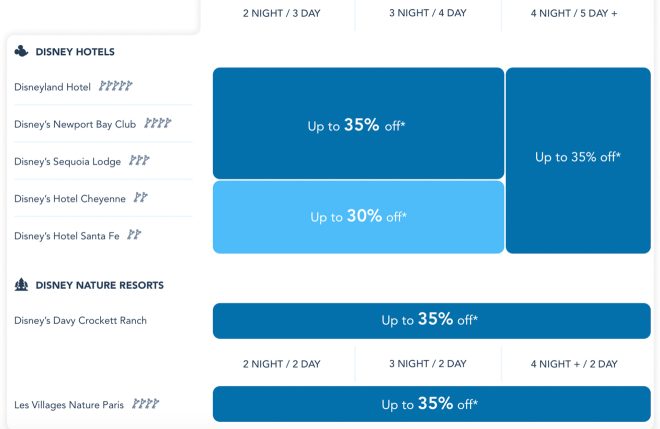The image is a screenshot of a Disney Hotels website featuring various accommodation options and special offers. On the left side of the site, there is a section labeled "Disney Hotels," complete with a rating system that seems to use either stars or Mickey icons, though it is not entirely clear. Below this heading, the hotels are listed with their respective ratings:

1. **Disney's Newport Bay Club**: 4 icons indicating a high-quality rating.
2. **Disney's Sequoia Lodge**: 3 icons indicating a moderate rating.
3. **Disney's Hotel Cheyenne**: 2 icons indicating a fair rating.
4. **Disney's Hotel Santa Fe**: 2 icons, similar to Hotel Cheyenne.

Additionally, the site mentions **Disney Nature Resorts** such as **Disney's Davy Crockett Ranch** and **Villages Nature Paris**, each with their respective ratings.

On the right side of the webpage, there are options for vacation packages, listed by duration at the top: "2 nights 3 days," "3 nights 4 days," "4 nights 5 days," and "5 days and more." Below these options, there are promotional buttons highlighting discounts of up to 35% off for various lengths of stay. The clickable elements on this side are mainly shaded in blue, while the background of the website is predominantly white.